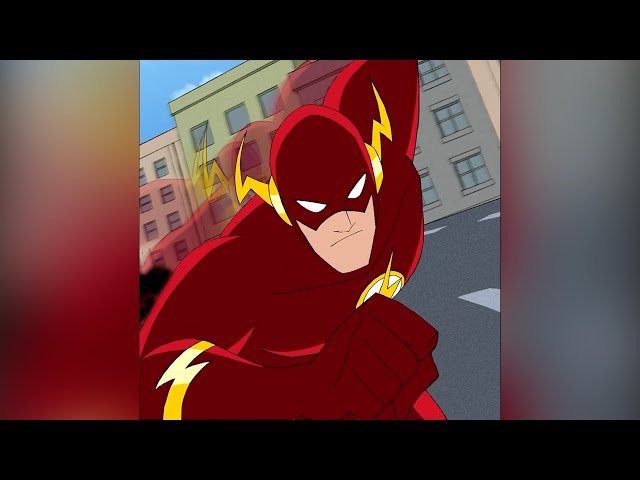The image is a detailed screen grab from a cartoon of the DC superhero, The Flash. The picture features The Flash in his iconic red costume with gold accents, including ear cups adorned with yellow lightning bolts that resemble horns. His mask covers his forehead and eyes, leaving only the whites visible, while his nose to chin area is bare, showing his light skin. The Flash's chest displays a circular emblem with a white background and yellow trim, featuring a yellow lightning bolt in the center. His suit also includes a prominent lightning bolt around his forearm.

The image emphasizes his dynamic motion, with a semi-transparent trailing effect of The Flash behind him, illustrating his incredible speed. His left fist is extended towards the camera, while his right arm is pulled back, enhancing the sense of swift movement. The background consists of gray buildings, a sliver of blue sky with white clouds, and the black surface of a city street below. The scene is framed by horizontal black bands at the top and bottom, and blurred wide bands on the left and right edges, further focusing attention on the clear central image of The Flash in action.